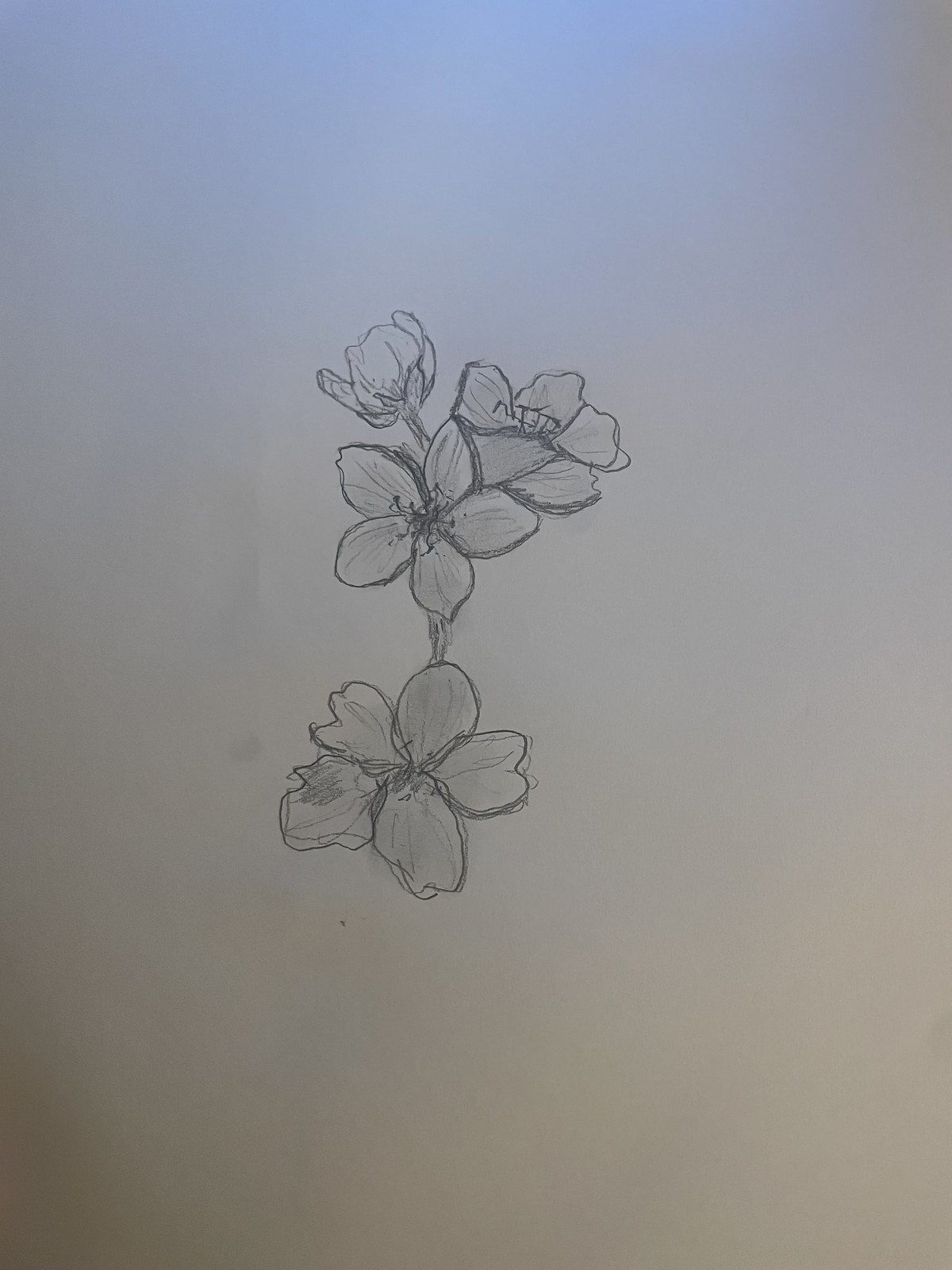The photograph captures a tall, rectangular piece of paper showcasing a detailed, hand-drawn pencil sketch of four flowers. This sketch, rendered in pencil with light shading and smudging, elegantly presents the flowers in a vertical arrangement. At the bottom, there's a single flower with five petals, connected by a stem to another flower above it. To the top left of this central flower, there is a budding flower, and to the right, a larger flower with open petals. The entire composition of these flowers is suspended in white space on the sheet, which features a light blue hue near the top, likely due to the camera flash. The paper is notably taller than average and may resemble tracing paper. It appears that the artist is practicing flower sketches, highlighting different petal architectures effectively.